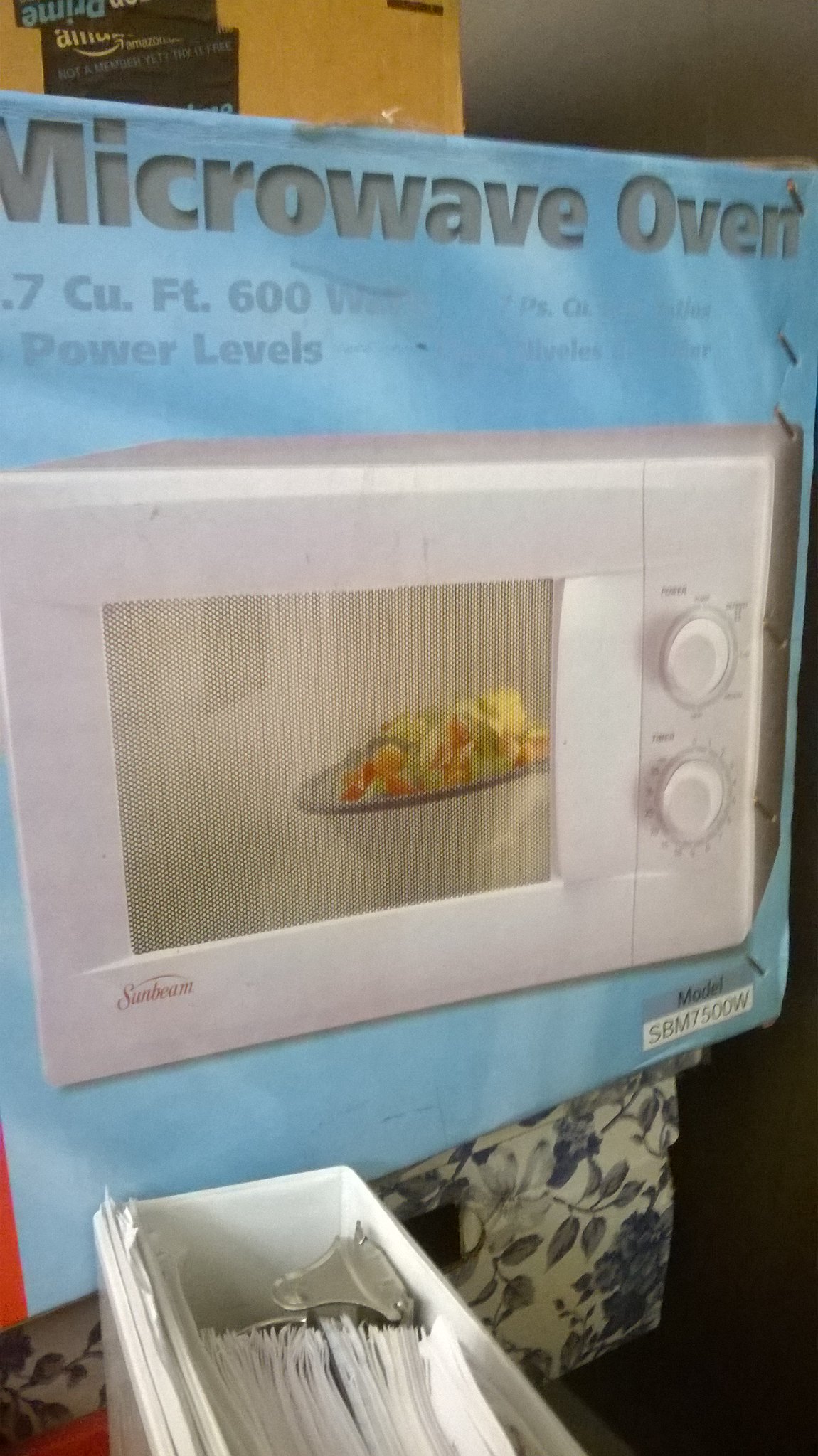The image captures a scene inside someone's house, prominently featuring a weathered blue microwave oven box with various details. The box, indicating specifications like "0.7 cu ft" and "600 watt power levels" in gray text, predominantly shows a silver Sunbeam microwave that has two large knobs on the right and the brand name on the left. Inside the microwave's central window, a colorful bowl of food, with visible red, green, and yellow items, can be seen heating. Below this box, a white binder is noticeably filled with a thick stack of papers, some fastened to the laminate front cover with a silver tab opening the binder rings. Another box with a blue floral print, visibly compressed under the microwave box's weight, is also in view. At the top of the image, an Amazon box with black Amazon tape spans across, adding to the layered and cluttered domestic environment.